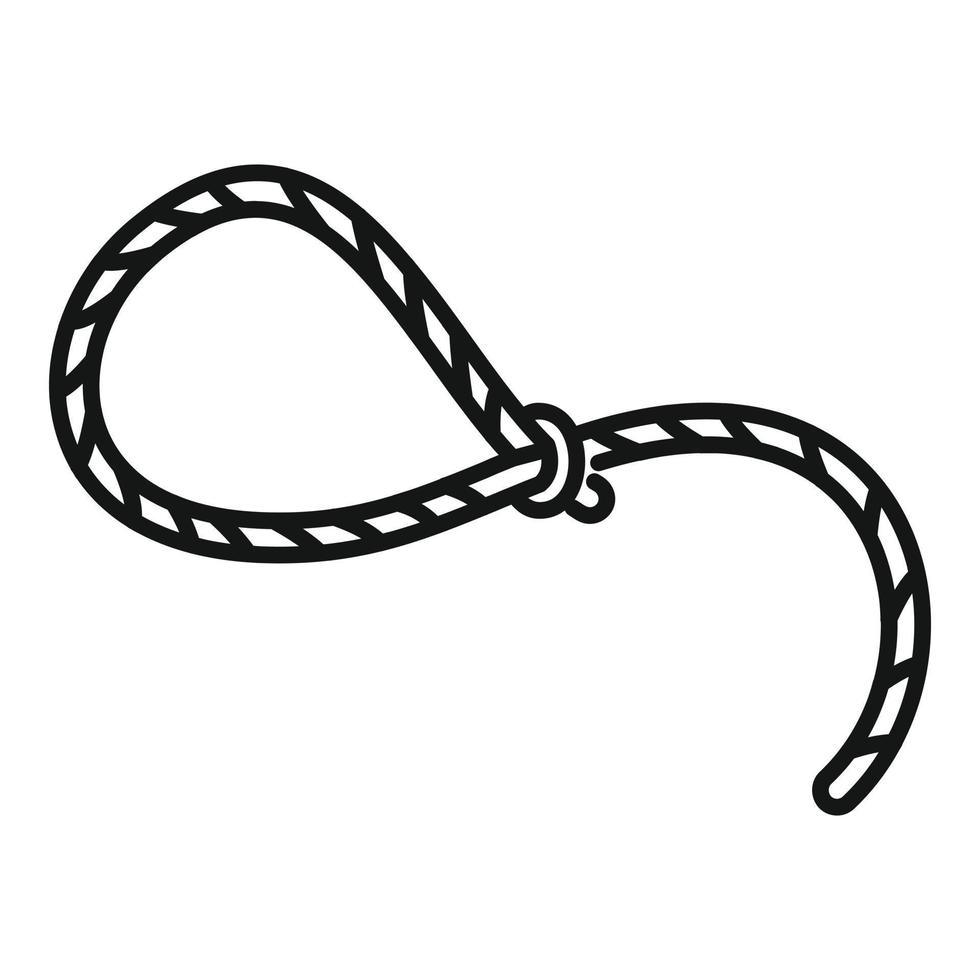The image is a simple, black-and-white drawing rendered with thick lines, resembling a broad-tipped pen or sharpie marker. It features a single, looped rope, similar to a slipknot or lasso, with the end of the rope extending to the bottom right of the image. The left side of the knot is tied together, forming an S shape that leads into a loop. The design of the rope appears braided, broken into segments, and tied together with a band, giving it a noose-like appearance. The background is entirely white, with no additional elements, text, or figures, making it a straightforward and easily replicable illustration.